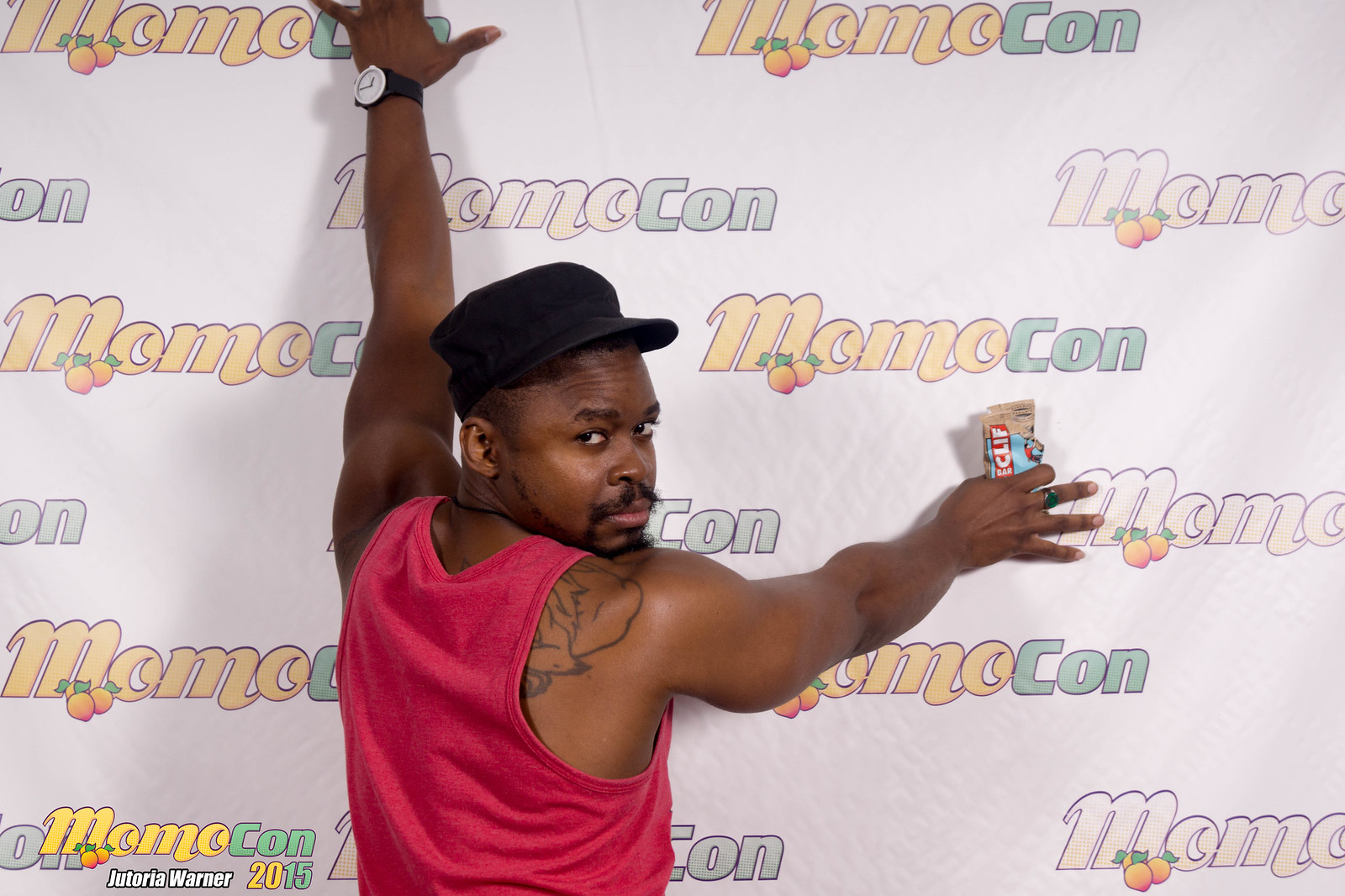In this vibrant image, a man strikes a dynamic pose with a product held in his right hand. His back is to the camera, yet he has turned his head around, giving the viewer a glimpse of his face. He is notably wearing a black cap and an eye-catching tank top that is a red hue, verging on pink. His left wrist is adorned with a sleek black watch, while his right hand, which also sports a ring, is in contact with a wall. The wall prominently features a banner for MomoCon, an annual multi-genre convention held in Georgia. In the lower left corner of the image, the MomoCon 2015 logo is clearly visible, along with the name "Jutoria Warner," possibly referring to the person in the image or an associated individual. The scene captures both the energy of the event and the stylish details of the man's attire and accessories.